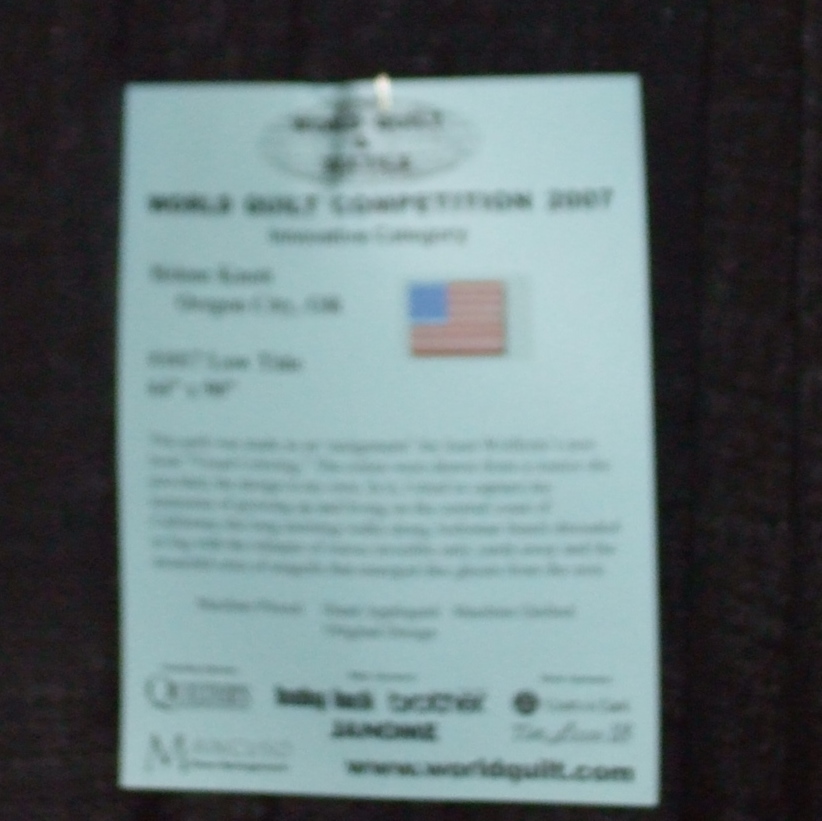This close-up photograph captures a very grainy and blurry piece of paper tacked to a dark surface, possibly a wall or pole. The paper features an American flag in the upper right-hand corner, about a third of the way down. Below the flag, there's a sizable, albeit unreadable, paragraph of text, indicating it might be a letter or notice. The text is in black font, interspersed with some thicker, bolded sections. At the top of the paper, there are dates and some partially discernible words, including "world" and "certification, 2007," though much of it remains illegible. The paper appears to be secured by a white thumb tack or hook, and at the bottom, there are multiple signatures and logos, though they are too blurred to read clearly. An oval shape at the very top near the thumb tack contains additional text. Despite the poor quality, a website address is faintly visible at the bottom.